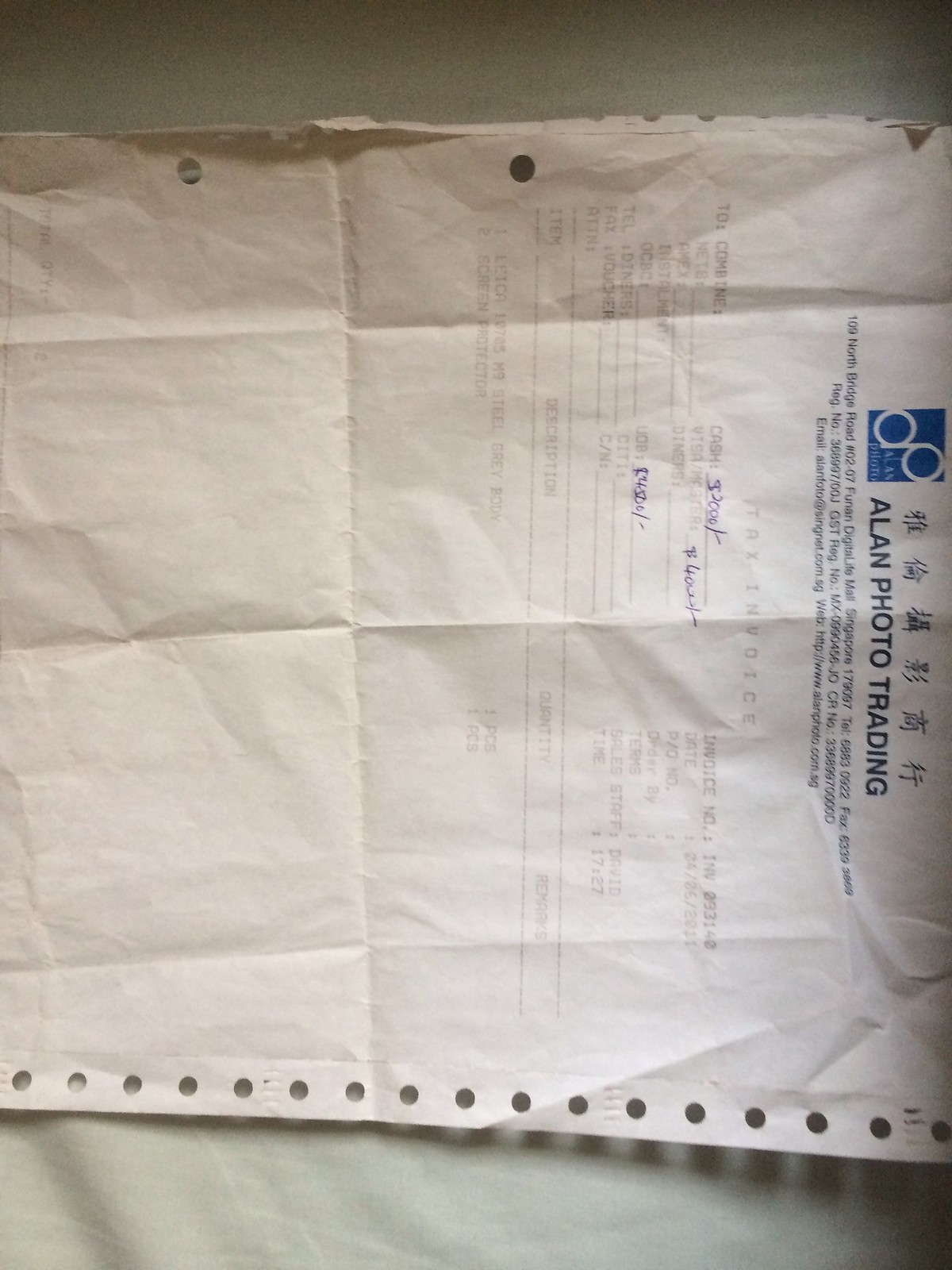A close-up photograph showcases an invoice document positioned against a white fabric backdrop. The invoice, predominantly white, prominently displays the text "Allen Photo Trading" in bold black lettering centered on the sheet. To the left of this title, a blue square features an intertwined "D" and "P" symbol, rendered in white. Beneath "Allen Photo Trading," there is additional black text that is blurred and unreadable, followed by the clearly visible gray inscription "Tax Invoice." A blue pen signature marks the document, though the signature and further details of the invoice are obscured by blurriness. Evident folding and slight crumpling suggest the invoice had been compacted in someone's pocket.